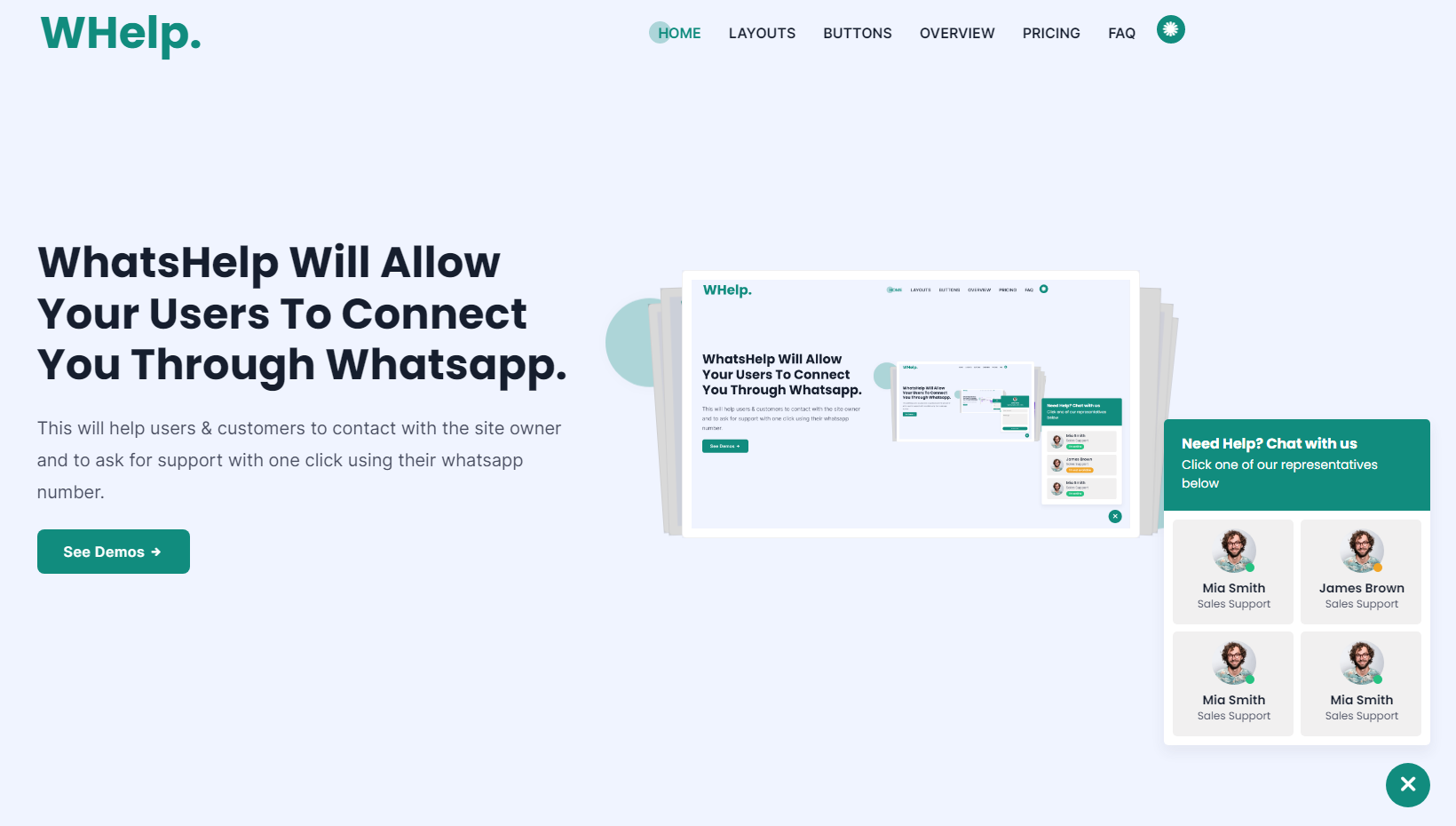This image is a cropped screenshot of the desktop homepage for a website named "WHELP." In the top-left corner, the WHELP logo is prominently displayed in dark blue. Towards the right side of the header, there is a horizontal list of categories in small gray font, including "Home," "Layouts," "Buttons," "Overview," "Pricing," and "FAQ." There is also a small green circle with a white dot in the center positioned in this section.

The background of the page is a light green color. Centrally positioned on the left side of the page, there is a bold, large-text section that reads, "WHELP will allow your users to connect with you through WhatsApp." Below that, there is a smaller text block explaining, "This will help users and customers to contact the site owner and ask for support with one click using their WhatsApp number." Directly beneath this text, a prominent green button labeled "See Demos" invites users to explore further.

To the right of the informational text, there's a mockup image displaying a WhatsApp interface. Further to the right, there is a square image of a "Need Help? Chat With Us" box, which features four profile pictures of support help desk staff, suggesting available customer service representatives ready to assist.